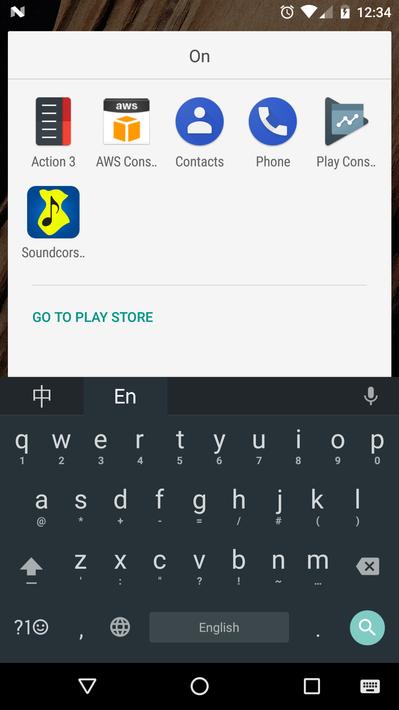In this screenshot, the image is vertically elongated with a black background. At the upper right corner of the top header, there are icons indicating a lit Wi-Fi signal, a full battery, and the time reading 12:34. Centrally located in the window is a white box with several elements inside it. From left to right, it reads "Action 3" accompanied by an icon of a black paper above the text.

Next to it, there is an "AWS" section featuring a distinctive white and black box with an orange cube at the center. Moving to the right, the text reads "Contacts," followed by "Phone," and "Play." Below the "Action" icon, there's another square icon, this time blue, with a music note symbol inside it, labeled "Sound Course."

Directly beneath these icons, in green text, there is a prompt that says "Go to Play Store." At the bottom of the image, the keyboard is visible with a black background, displaying keys with white letters.